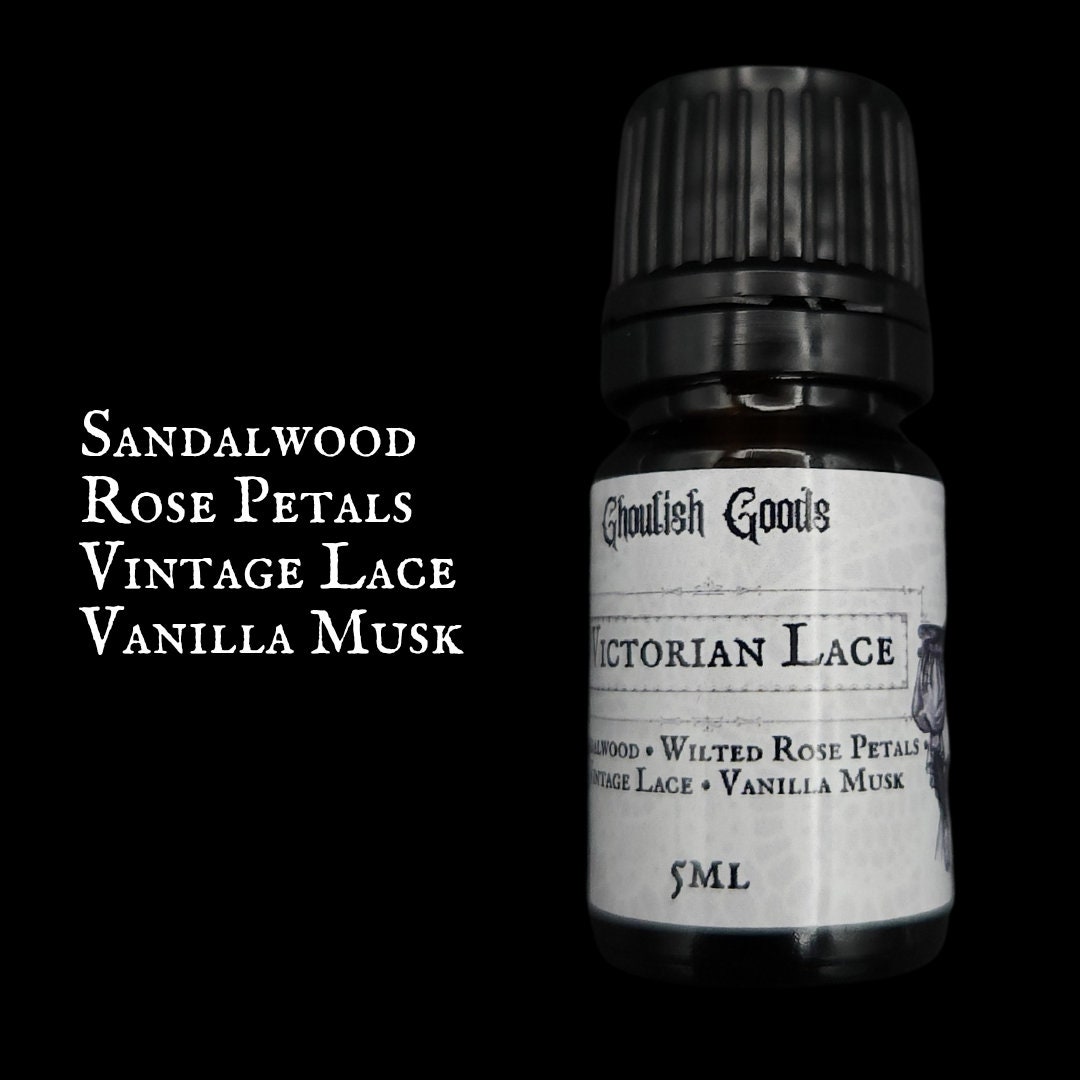The image showcases a close-up of a small, black, glass bottle with a black, plastic, grooved cap, set against a black background. The bottle features a white label with black text in an old-timey font, exuding a vintage apothecary aesthetic. Prominently displayed on the label are the words "Ghoulish Goods, Victorian Lace" along with the details of the essential oil blend: Sandalwood, Wilted Rose Petals, Vintage Lace, and Vanilla Musk. The bottle has a capacity of five milliliters. An additional image or illustration is partially visible towards the side of the label. The overall presentation suggests an air freshener or perfume, reminiscent of an old-fashioned product, though recently crafted to appear antique. The black and white color scheme, coupled with the reflection on the bottle from the camera flash, enhances the classic, nostalgic appeal.